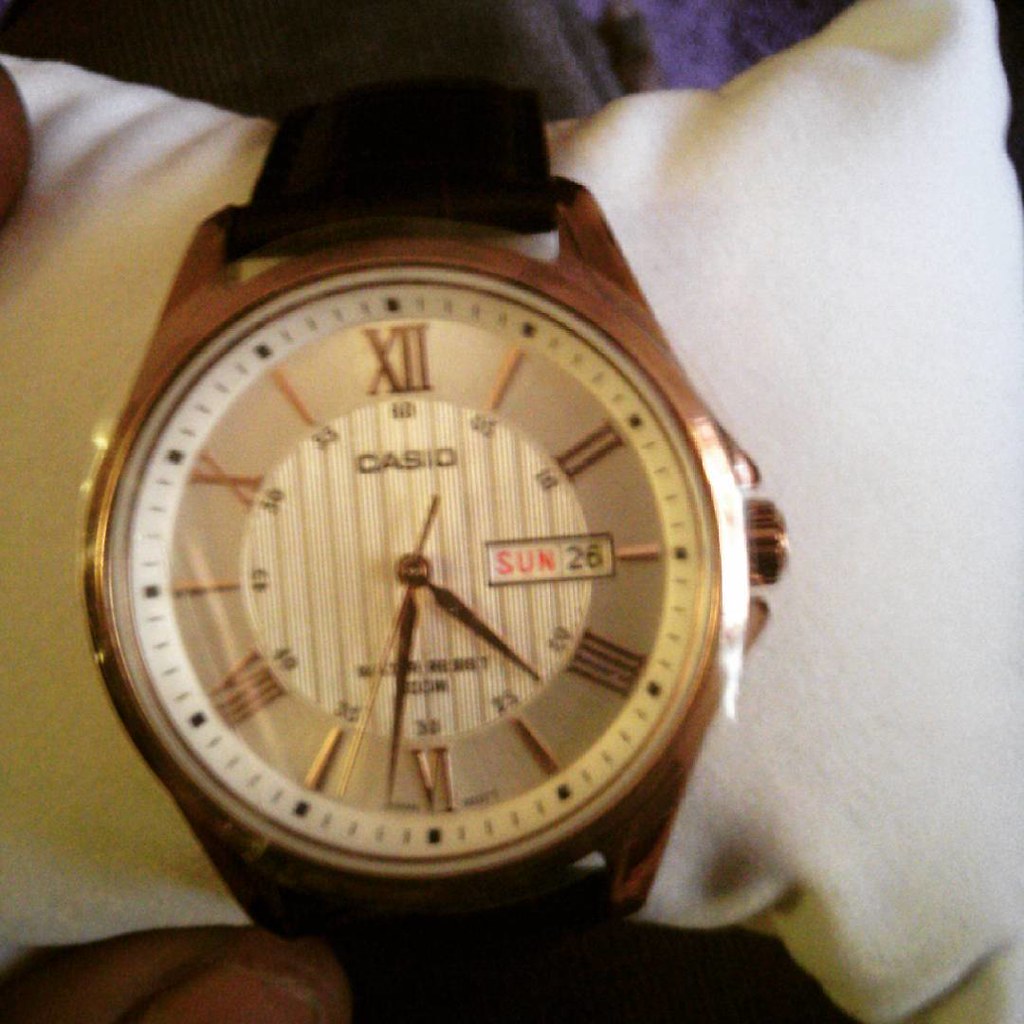In the photograph, a wristwatch is prominently displayed, seemingly prepared for sale or kept in storage. The watch is attached to a white pillow, which helps maintain its shape. Despite the slight blurriness of the image, details of the watch can be discerned. The watch features a black band that appears to be made of leather. Its housing is either gold or a copper hue, adding a touch of elegance. The watch face is silver and adorned with gold Roman numerals, enhancing its classic aesthetic. The brand name "Casio" is clearly visible on the face, indicating the manufacturer of this timepiece.